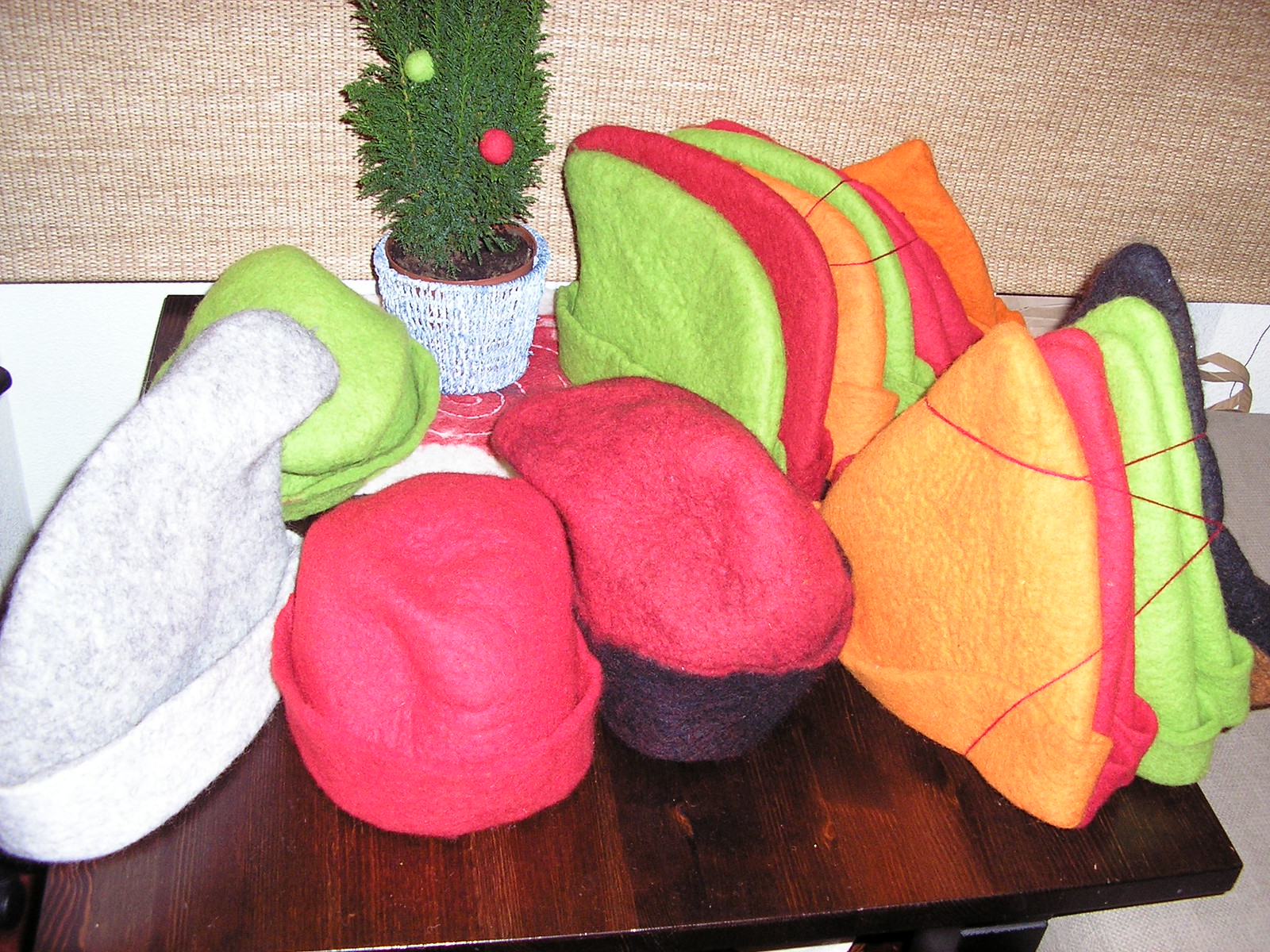This indoor color image captures a cozy Christmas-themed arrangement featuring a small, square-shaped dark brown wooden table set against a white wall with a brown curtain-like shade above a window. On the table sits a white pot, adorned with a crocheted cover, holding a small green plant that appears to be a lemon cypress tree or a similar small tree. Embedded in the soil are two spherical ornaments, one red and one apple green, reminiscent of Christmas decorations.

The table is also adorned with various handmade felt hats, which appear to be wool or craft felt. These hats vary in shape and color, predominantly featuring winter cap styles. Two distinct piles of hats stand upright, with their open ends on the table. One pile includes hats with pointed tops, while the other has rounded tops, both tied together with red string. Additionally, individual hats, thicker in fabric, stand separately on the table, displaying colors such as green, pinkish, orange, reddish, white, black, yellowish-gold, and gray. The scene evokes a festive, handmade charm, suggesting the hats might be elf hats or part of a whimsical holiday display.